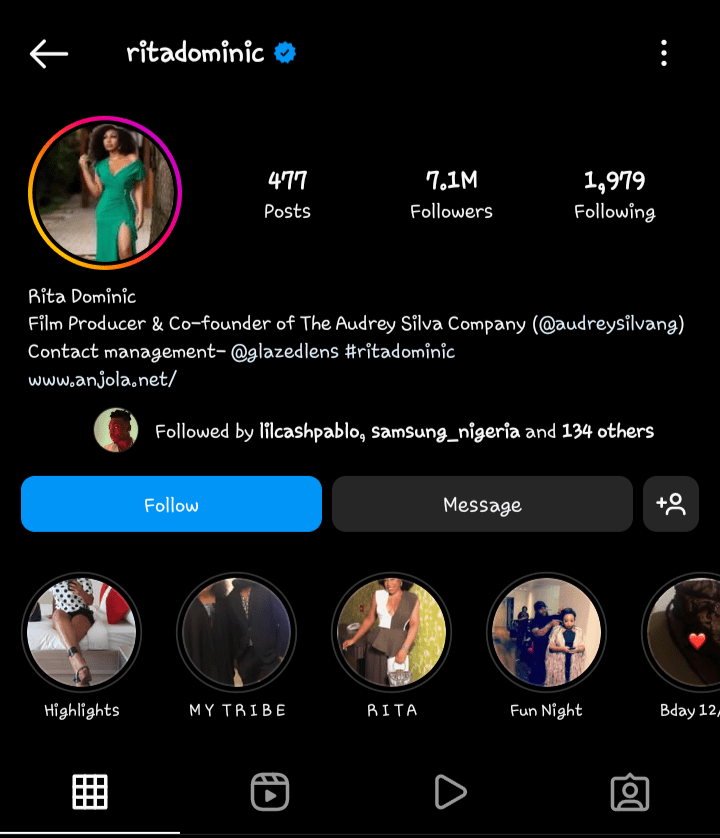The image features a stark black background. In the top upper left corner, a white arrow points to the right, next to which is written "RITA DOMINIC" in uppercase white letters. A blue circle bearing a black checkmark appears beside her name, indicating a verified profile.

Beneath this, there is a circular profile picture showcasing a woman in a green dress, visible down to just past her knees. She has long, dark, shoulder-length hair and is facing forward while holding one arm up. Adjacent to the profile picture, text reads: "477 posts, 7.1 million followers, 1,979 following."

Following this, a descriptive paragraph states: "Rita Dominic, film producer and co-founder of The Audrey Silva Company. Contact management."

Below the paragraph, a smaller circle displays the face of a man, accompanied by the text, "Followed by LilCashPablo, Samsung_Nigeria, and 134 others."

At the bottom, a blue bar with the word "Follow" sits in the center next to a gray bar with the word "Message." Below these bars, there are additional circles featuring images of various people, each accompanied by their respective usernames.